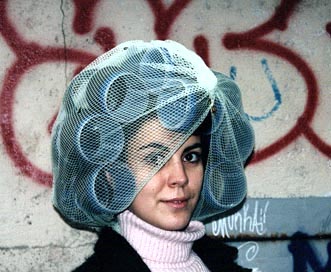In a photograph reminiscent of the 1980s, a young woman in her mid-to-late 20s poses confidently. She stands against a gritty backdrop featuring a white cement wall adorned with vibrant red bubble-letter graffiti. Her attire consists of a pink turtleneck layered under a dark jacket. Her hair is meticulously styled in large light blue curlers, approximately three inches in diameter, fully wrapped in a white, translucent hair net designed to hold the curlers in place. The scene captures an intriguing blend of retro fashion and urban elements.